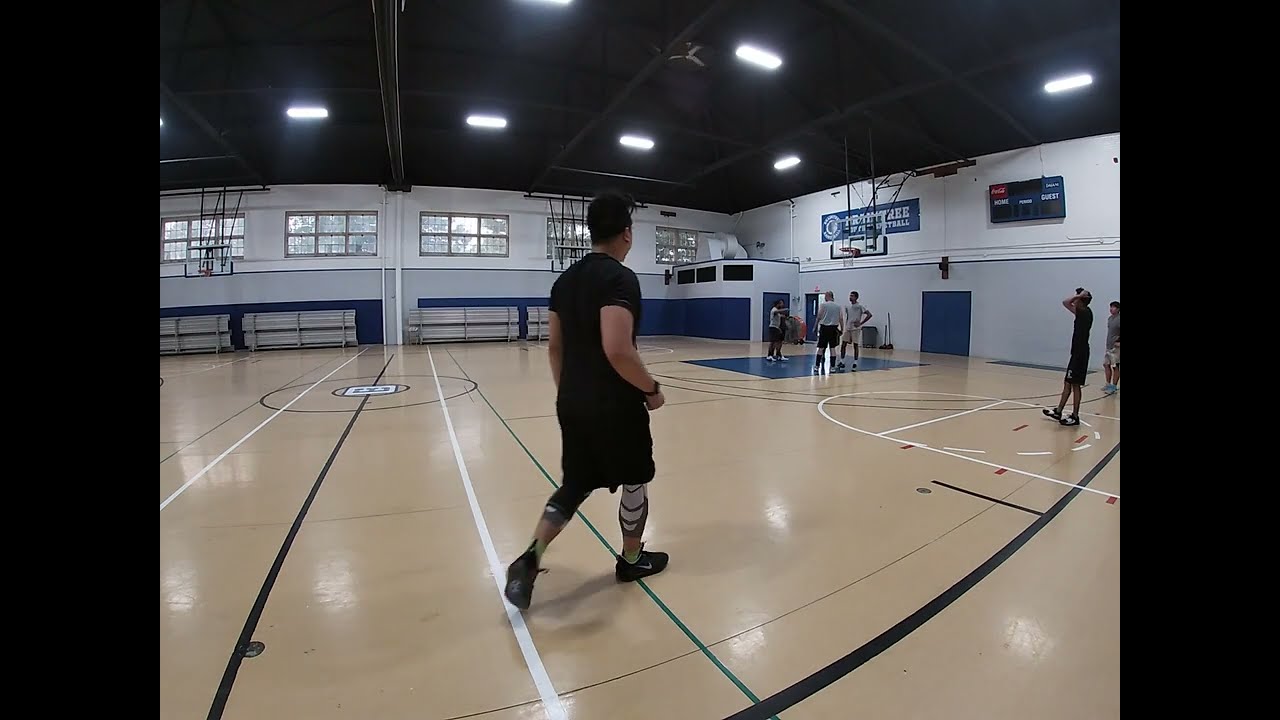The image captures an indoor basketball court, showcasing a large gymnasium with white and gray walls. In the foreground, a man dressed in a black t-shirt, black basketball shorts, and black Nike shoes with white swooshes stands with his back to the camera. He appears to be moving past the half-court line, wearing compression socks or knee sleeves. The shiny, light brown basketball court reflects the ceiling lights, and there are black, white, and green lines marking various areas on the floor. The gym features a tall ceiling adorned with large lights and banners around a scoreboard near the basket. Several other people in casual clothes—shorts and t-shirts—are scattered around the court, especially under the basketball hoop and to the right. Bleachers, likely pushed back, are visible at the far end, and above them are windows that let light into the space. There's a door located in the far right of the image.